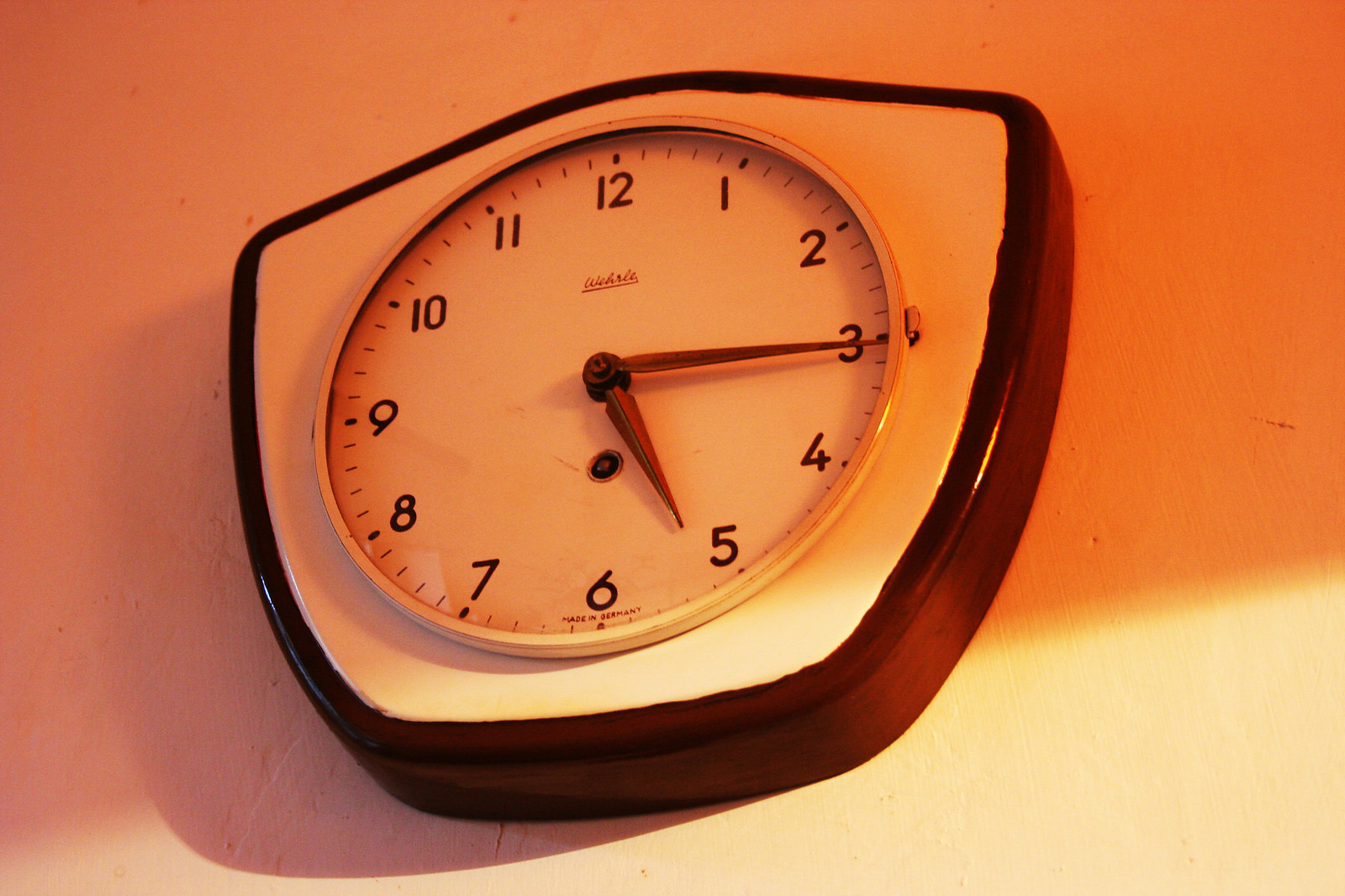The image depicts a vintage wall clock mounted on a wall that has a faded cream or brownish-pink hue. The wall is illuminated by a light source, possibly sunlight, giving it a subtle orange tint and casting a distinct shadow from the clock. The clock's frame is dark, either black or dark brown, with a unique design where it curves up at the top and narrows slightly towards the bottom. The clock face is a weathered white, indicating its age, and is encircled by a white border. Clear, black numerals mark the hours, and the hands, one large and one small, are brown. The clock reads approximately 5:15, with the minute hand on the 3 and the hour hand on the 5. Beneath the 12 o'clock position, there seems to be a brand name in a script font, possibly underlined, but it is too faint to discern clearly.